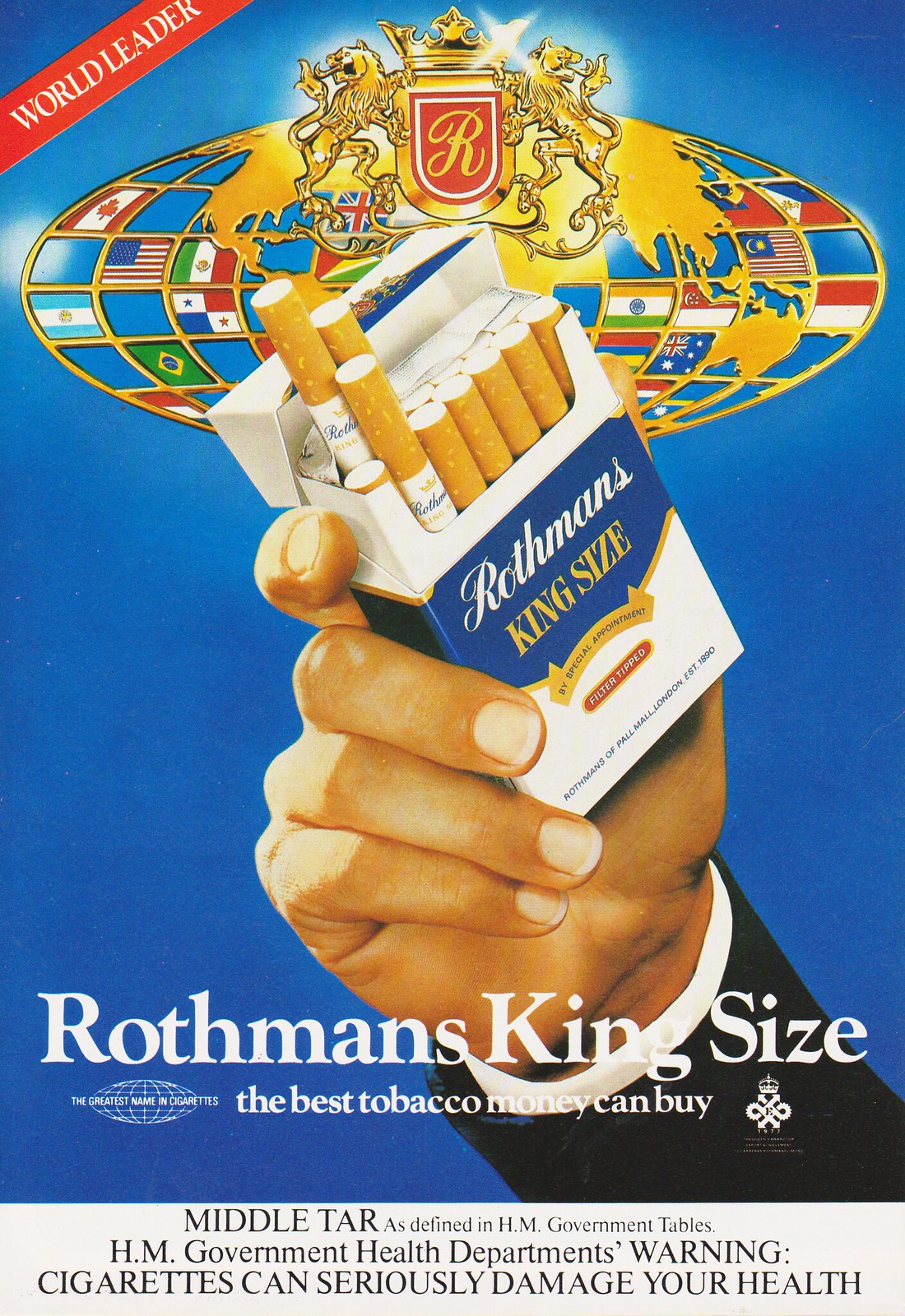The advertisement is a vertical, rectangular image showcasing Rothmans King Size cigarettes against a blue background. Central to the image is a white pack of cigarettes with two or three filters partially visible, held by a man whose manicured hand emerges from the bottom right corner. Over the pack is the brand's distinctive coat of arms, featuring a red shield with a golden 'R' and flanked by lions, topped with a crown. Above this is a globe composed of multiple flags, symbolizing international presence, and a red diagonal banner in the top left corner reads "World Leader" in white text. The package has a blue label with "Rothmans" in white script and "King Size" in gold beneath it. At the bottom, bold text declares, "Rothmans King Size: The best tobacco money can buy," flanked by white logos, one of which reads "The Greatest Name in Cigarettes." A health warning at the footer, in black text on a gray strip, states, "Cigarettes can seriously damage your health."